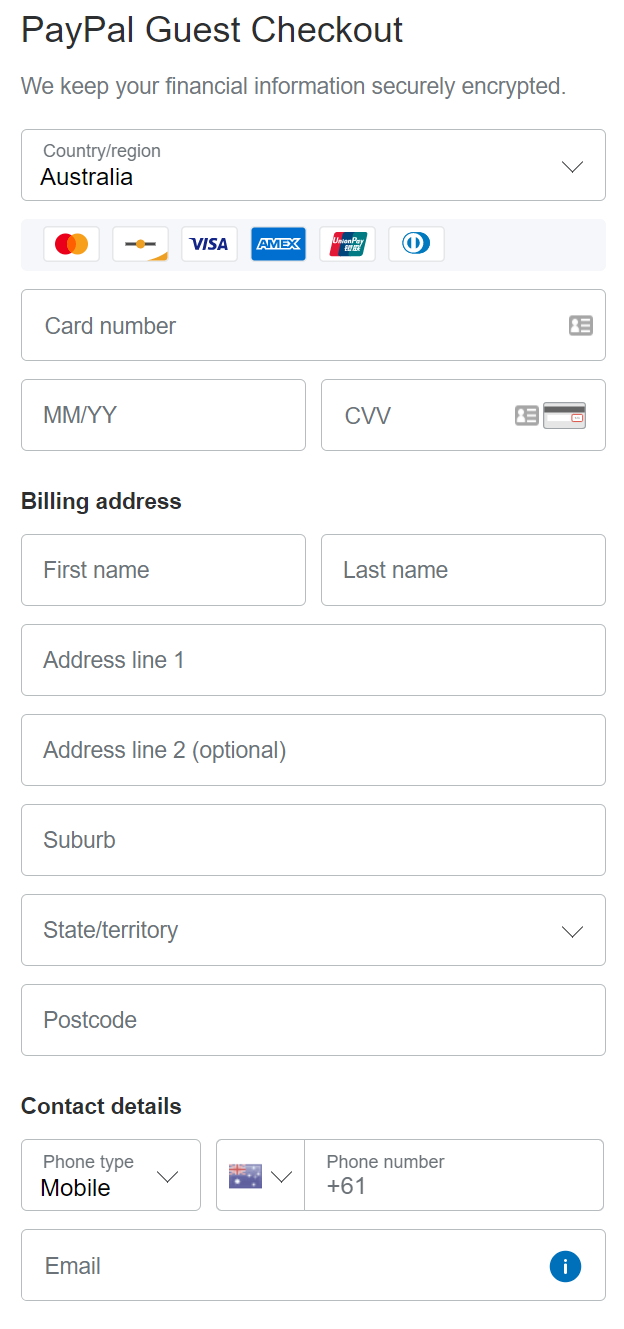The image showcases a screenshot of a PayPal guest checkout webpage displayed on a white background. At the top of the screen, the page title "PayPal Guest Checkout" is prominently displayed in black text. Directly below this, there's a message assuring the user that "We keep your financial information securely encrypted."

The form begins with a dropdown labeled "Country/Region" pre-filled with "Australia," followed by icons indicating accepted payment methods, including MasterCard, Visa, AMEX, and several other card types.

Next, there are fields to input card information: "Card Number," "Expiration Date" labeled "MM/YYYY," and the "CVV Number." Below these, there are sections for billing address details containing fields for "First Name," "Last Name," "Address Line 1," and an optional "Address Line 2." Additional fields request information for "Suburb," "State/Territory," "Postcode," and "Contact Details," specifying the "Phone Type" as "Mobile."

Centrally positioned is an image of a payment card. To the right of this image is a box labeled "Phone Number," pre-filled with the country code "+61" for Australia. Beneath this is an "Email" field, which features an icon of a blue circle with an eye symbol on the right-hand side, hinting at a feature to reveal the email input.

The entire webpage is neatly structured against a clean, white background, emphasizing the user interface's clarity and ease of use.